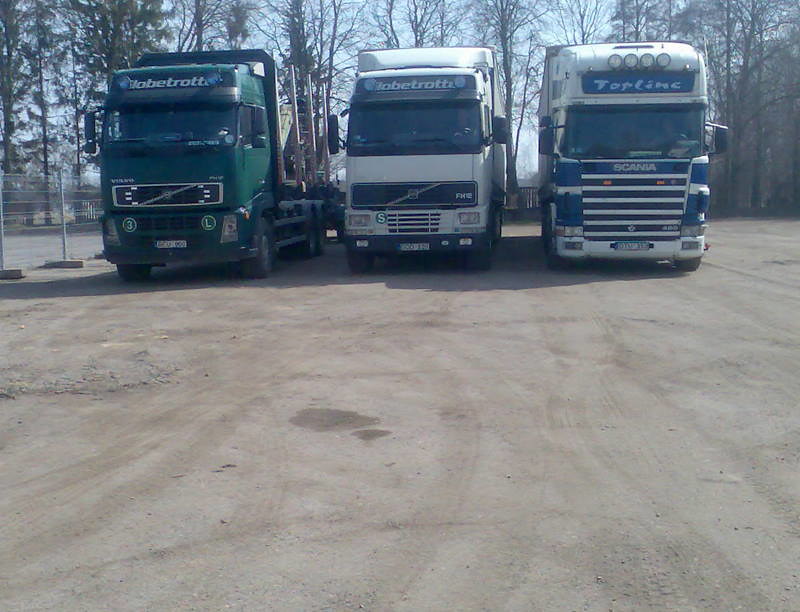This color photograph captures the front view of three large trucks parked side by side in a lot. The trucks are situated on a grey, dusty surface with thin tracks visible, suggesting a well-traversed area. A wire fence is visible to the left of the image, enclosing the space. The green truck on the left is a Volvo with the word "Globetrotter" written above it. The middle truck appears silver-yellow and also has "Globetrotter" along with "FFHE" visible on its front. The third truck, on the far right, is blue and white, with "Scania" and "Tour Line" marked on its front, and it also features an additional row of lights above the brand name. Behind the trucks looms a line of barren trees, indicating a winter scene, under a greyish blue sky. The setting appears to be a spacious, open lot amidst an incomplete, leafless forest.